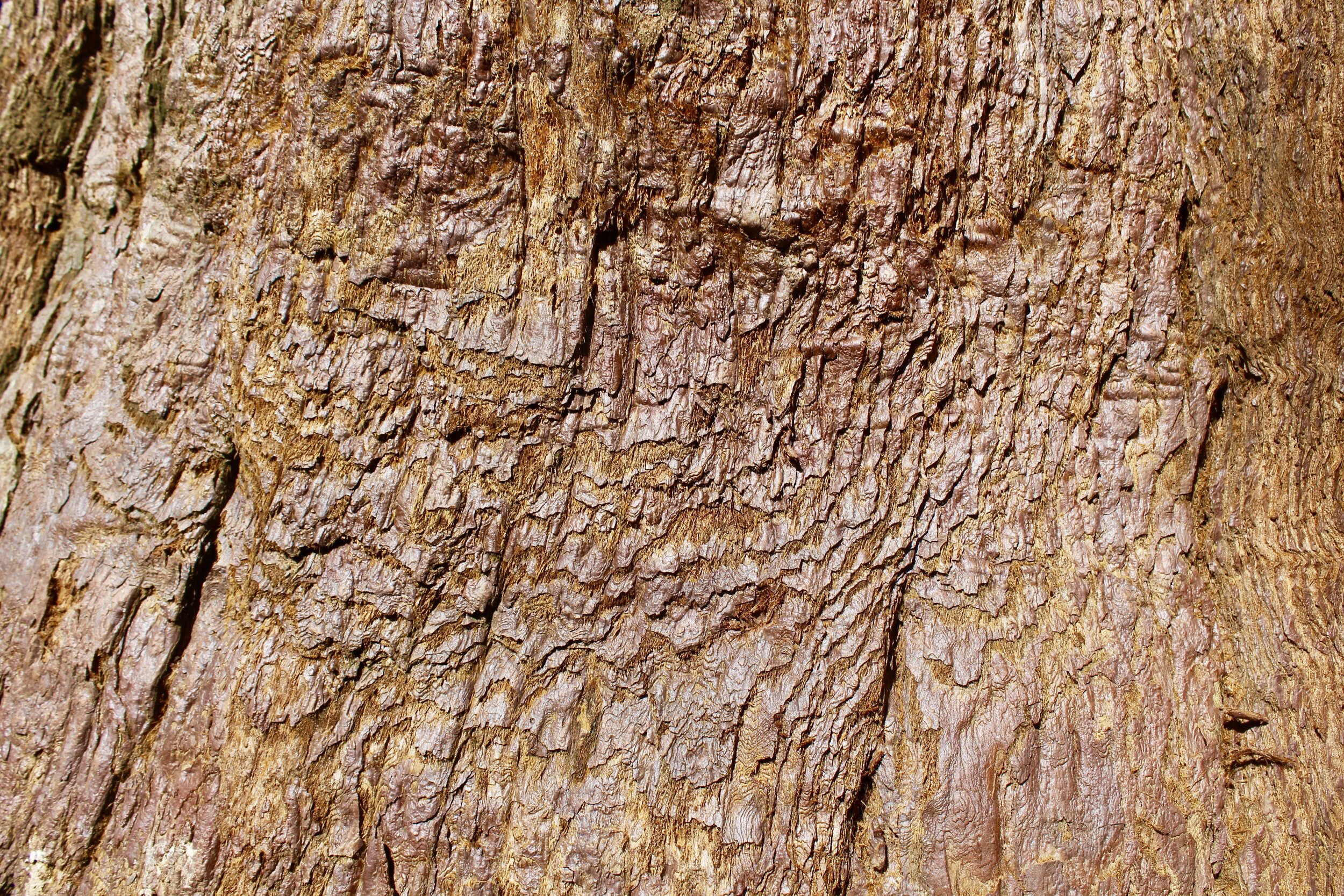The photograph is a heavily zoomed-in, detailed close-up of a natural surface, likely the bark of a tree or a rocky texture that closely resembles the appearance of bark. The surface is gnarled with numerous ridges, curves, nooks, and crannies, creating a complex and intricate landscape. The primary color is a gray-brown, interspersed with darker patches that appear to have been stained by water, adding a varied texture to the image. Scattered across the surface, there are spots of green vegetation, suggesting some plant life is thriving on this rough terrain. The surface appears slightly sloped and exhibits a mixture of smooth, shiny areas alongside rough, cracked patches. The image is uniformly focused on this textured field, with no other features visible outside the frame.